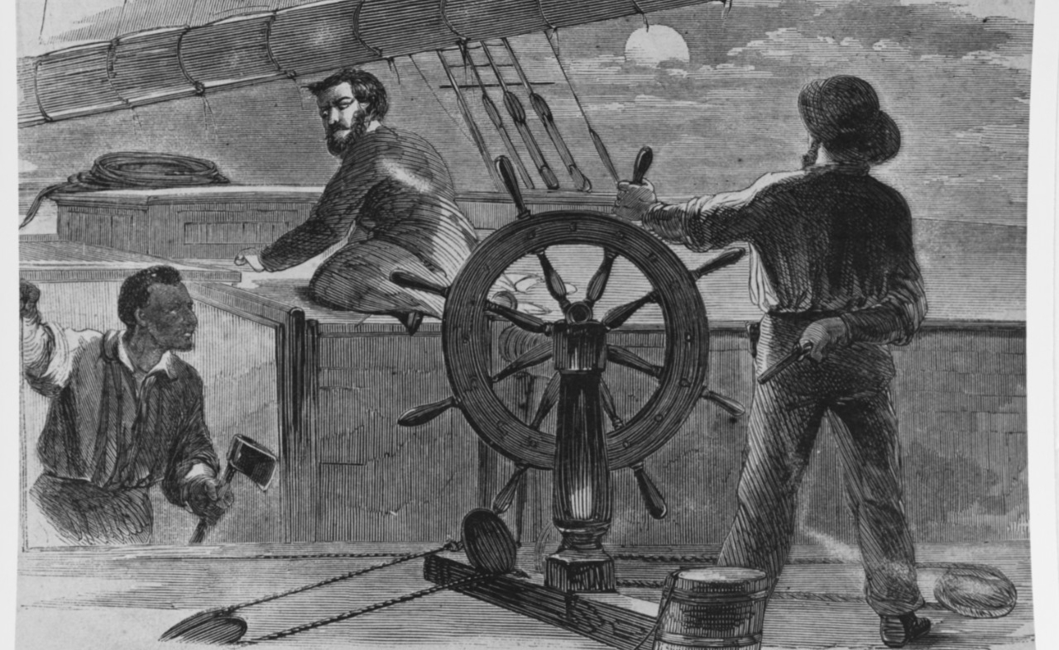This detailed black and white sketch, possibly created using pencil or charcoal, captures a tense moment unfolding on a historical ship. The central figure, a man in a flowy blouse and pants, stands with a wide stance at the ship's wheel. His left hand grips the wheel while his right hand is concealed behind his back, possibly hiding a weapon like a gun or a knife. In the lower left, a darker-skinned man ascends from below deck with an axe in his left hand and a loose-fitting blouse, gripping the ship with his right hand for balance. He appears to be moving toward a third man, who is seated on an elevated platform or a box to the right, gazing intently at the man climbing up. This bearded man with dark hair wears a tuxedo-style coat, hinting at an era possibly in the late 1700s or 1800s. The background features sails and rigging, with a partially obscured moon or sun peeking through the clouds, indicating a night scene. The overall composition suggests a possible mutiny or impending confrontation, with the atmosphere of the drawing accentuated by its stark, dramatic contrasts between black and white.